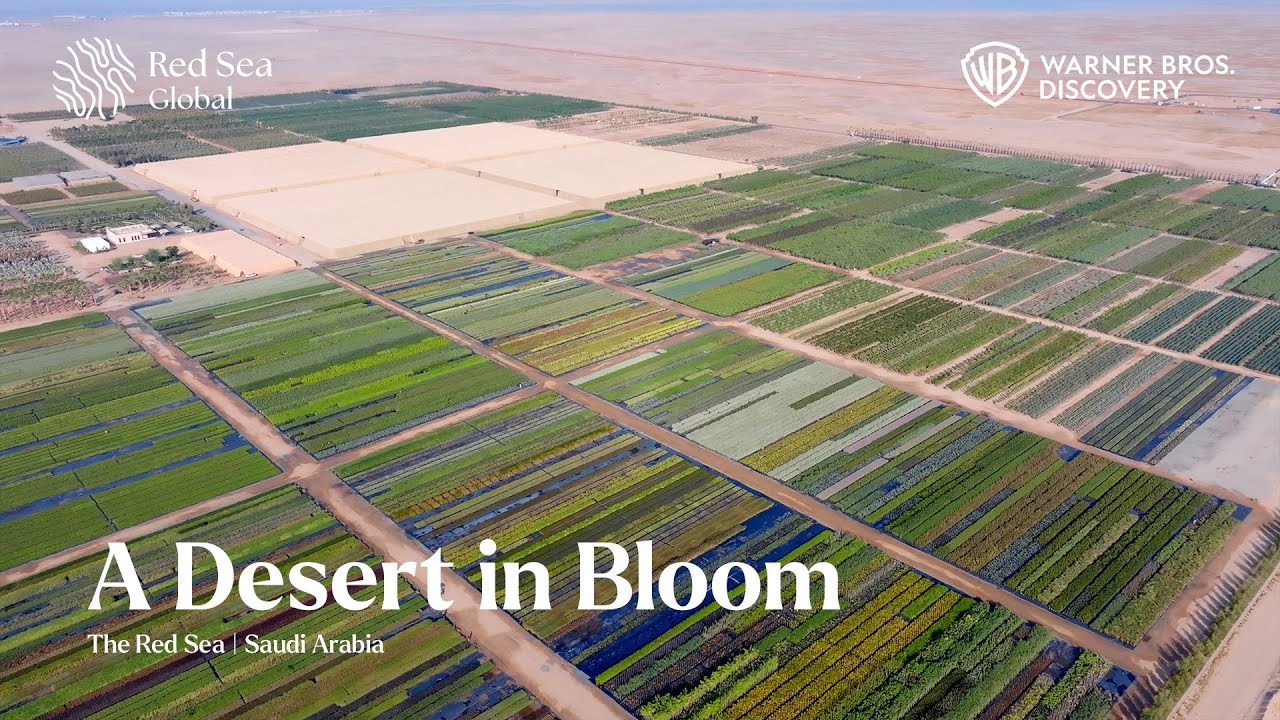This vibrant, marketing photo is an aerial shot taken in Saudi Arabia. It showcases four large, perfectly arranged white squares, surrounded by an impressive display of crops and vegetation in sprawling rows, featuring a mix of green, brown, and even some blue hues. The background extends into a vast, tannish-red desert, emphasizing the contrast with the blooming landscape. In the upper left corner, the text "Red Sea Global" is situated alongside a circular, squiggly emblem, while the upper right corner bears the Warner Brothers Discovery shield and text. The bottom left corner prominently displays the phrase "a desert in bloom" in large white letters, with "The Red Sea, Saudi Arabia" written just beneath it in smaller text. This horizontally rectangular, full-color image, enhanced for marketing purposes, powerfully illustrates the vibrant growth amidst the arid surroundings, symbolizing hope and transformation.